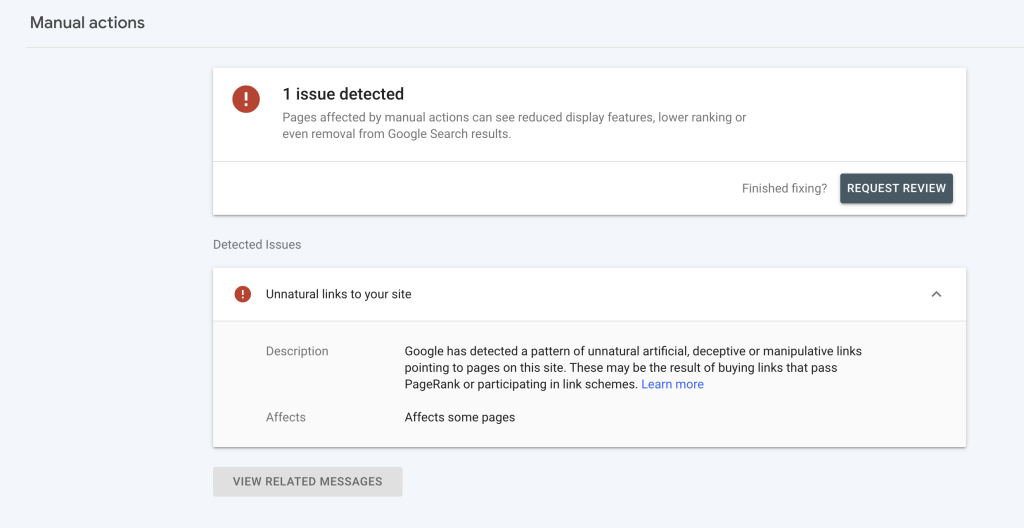The image is a screenshot from a website with an off-white background. In the top left corner, it features the text "Manual Actions." Below this, there is a large rectangle with a white background. In the top left corner of this rectangle, there is a red circle containing an exclamation point. Next to the circle, the text reads "1 issue detected." Beneath this, in smaller text, it states, "Pages affected by manual actions can see reduced display features, lower ranking, or even removal from Google search results."

In the bottom right corner of this rectangle, the text "Finished fixing?" appears, accompanied by a clickable button labeled "Request Review" with a darker gray background.

Further down, the text "Detected issues" appears, followed by another rectangular box featuring another exclamation point in a red circle. This is accompanied by the text "Unnatural links to your site."

Within this box, beneath the main heading, it reads "Description: Google has detected a pattern of unnatural, artificial, deceptive, or manipulative links pointing to pages on this site. These may be the result of buying links that pass PageRank or participating in link schemes." The phrase "Learn more" is highlighted in blue.

Continuing below, the text reads "Affects some pages," followed by a gray rectangular box saying "View related messages."